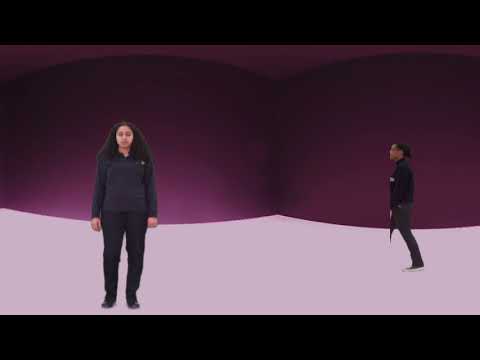The image depicts a three-dimensional, abstract pink room with curved walls and a distinctive contrast in tones. The back walls and ceiling are a dark plum purple, while the floor is a light lavender pink. Two people are present in this surreal space. On the left stands a medium-build woman with dark skin, shoulder-length wavy black hair, and closed eyes. She is clad in a black long-sleeve shirt, black pants, and black shoes. To her right is a man with dark skin and short black hair, walking from the right to the left. He is dressed in a long-sleeve black shirt, dark gray pants, and black shoes with white soles. The image is visually framed with black lines at the top and bottom, adding to the abstract nature of the setting.